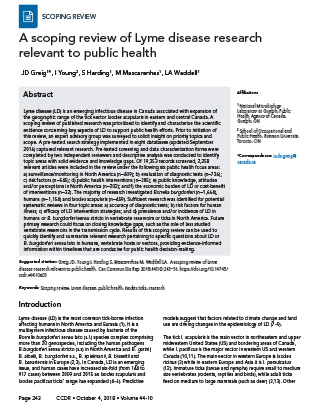The image depicts a screenshot of an academic article page. In the upper left-hand corner, there is a header that reads "Scoping Review." The article's title, "A Scoping Review of Lyme Disease Research Relevant to Public Health," is prominently displayed below. The authors' names are listed, but they are too pixelated to be legible. The background features a light gray rectangle, with the word "Abstract" in a larger font in the upper left corner. Below this header is a sizable paragraph of text in very small, unreadable print. Under the abstract, there appears to be a section likely dedicated to credits or affiliations. Following a noticeable break, the word "Introduction" signifies the start of a new section. The introduction text continues in a two-column format, with paragraphs extending from the left column to the right. The entire layout is set against a white background with black text.